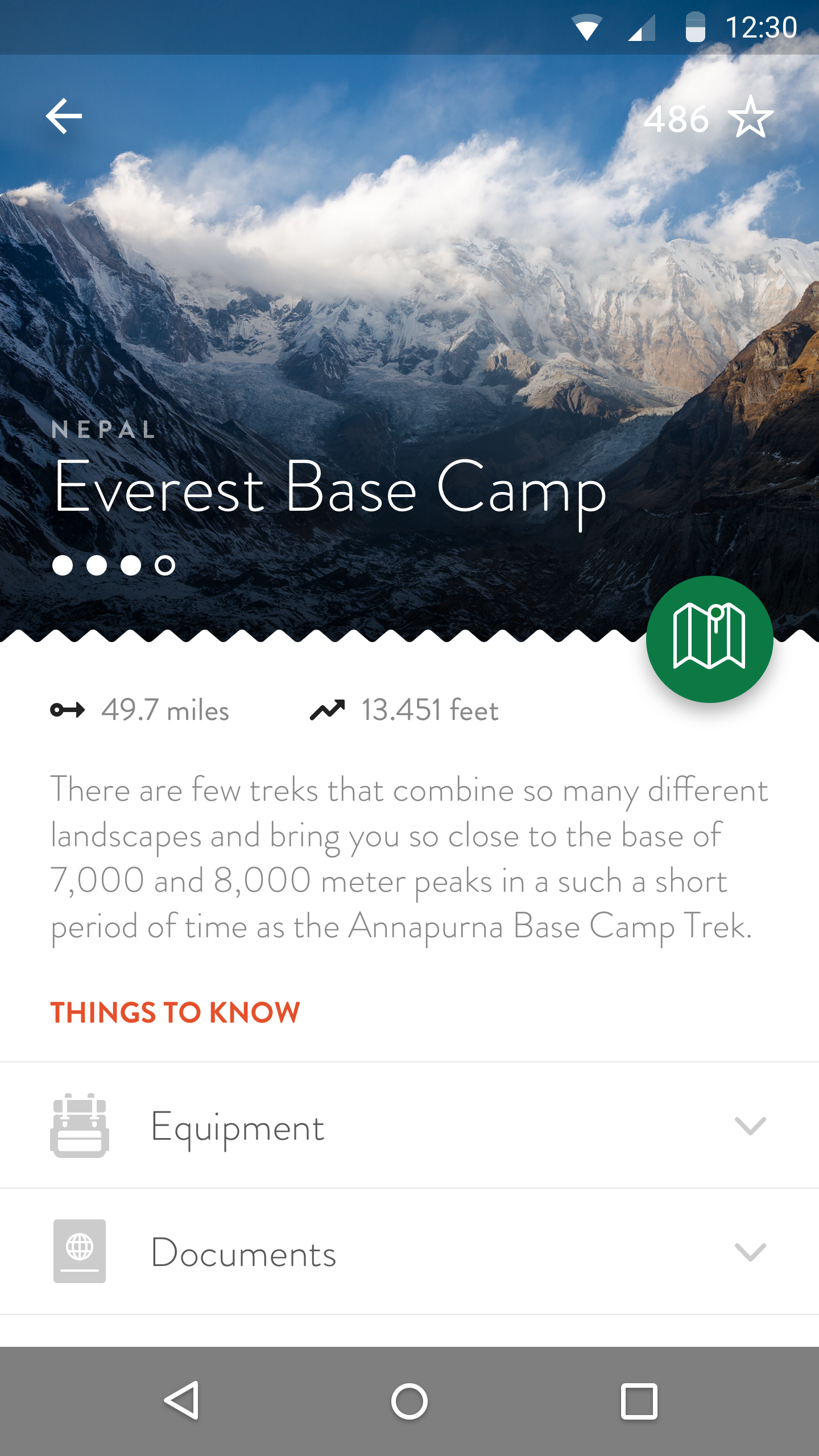The top portion of the screenshot, taken on someone's phone, features a blue border against a backdrop of a sky dotted with clouds. The image showcases a majestic mountain range, where the snow-capped peaks are vividly painted in white, while the exposed rocky areas reveal rugged terrain. In the foreground is a branch adding a natural frame to the scene.

At the top of the screen, the status bar indicates the time is 12:30. The phone’s battery icon shows less than 50% charge remaining. The cellular service appears weak, while the Wi-Fi connection is strong. On the left side of the screen, there's a white Apple logo pointing left, symbolizing the device's brand.

On the right side, it displays the number "486" and a white-outlined star. Below it, the text reads “Nepal Everest Base Camp,” accompanied by four circles—three filled in white, and the fourth only outlined. To the right of this, a green circle with a map icon is visible. Underneath, gray text states "49.7 miles, 13,451 feet," describing the trek's metrics.

A longer caption continues below the metrics:

"There are just a few treks that combine so many different landscapes and bring you so close to the base of towering 7,000 to 8,000 meter peaks in such a short period of time as the Annapurna Base Camp Trek.”

At the bottom, an orange notification mentions "Thanks" and "No," while in black text, it states "Equipment" and "Document."